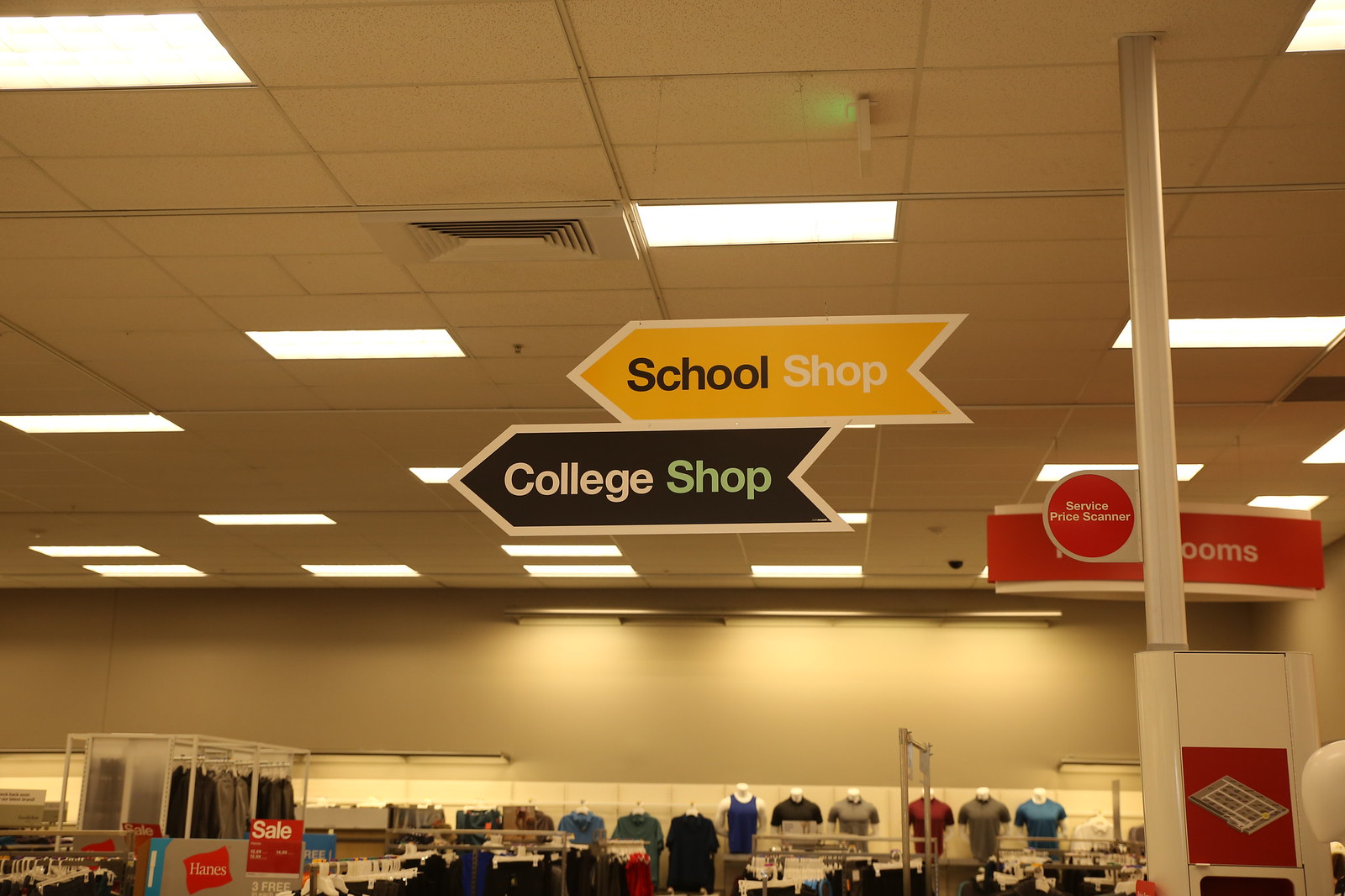The interior of a bustling retail clothing store is prominently featured in this image. The ceiling, fitted with drop panels and scattered with panel lights, provides ample illumination throughout the space. Suspended from clear wires in the center of the store are two directional signs. The top sign, a vibrant yellow arrow labeled "School Shop," points left, while directly beneath it, a black arrow marked "College Shop" also directs shoppers to the left.

In the background, a dual-toned wall is visible; the upper portion is painted gray while the bottom is white. Against this wall, several headless mannequins are dressed in various shirts, adding visual interest and showcasing the store's apparel. Additional shirts are neatly arranged on various racks and shelves throughout the store.

To the left, vibrant red signs indicate a sale, drawing customers' attention. Below these signs, an advertisement for Hanes is prominently displayed. On the right side of the image, a vertical pole features a red sign reading "Service Price Scanner," ensuring customers can easily check prices. The overall layout and signage guide shoppers efficiently through the store's diverse clothing sections.